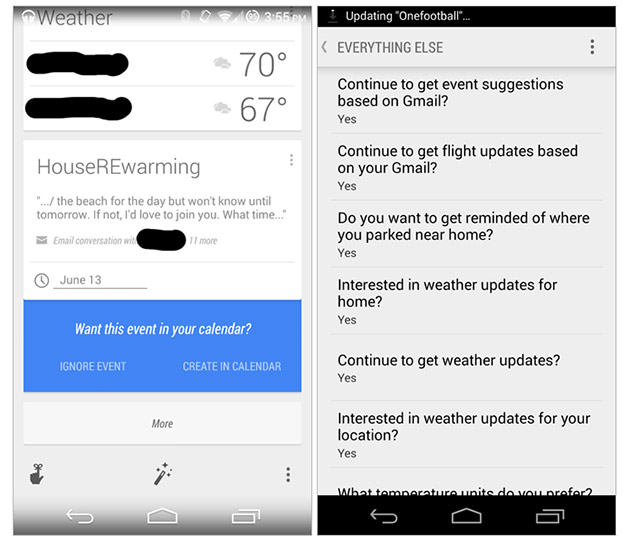The image consists of two equal-sized smartphone screenshots displayed side-by-side, forming a nearly square composition. Both screenshots showcase various app interfaces and notifications, providing a glimpse into typical smartphone usage.

On the left side, the screenshot appears to be from a weather application. At the top, the typical smartphone status indicators are visible, including signal strength and the current time, along with a few icons indicating active apps. Below this, the app header clearly displays "Weather," though specific locations are obscured, likely for privacy. The temperatures of 70°F and 67°F are shown beside respective cloud icons, suggesting current weather conditions. Additionally, there's a section labeled "House Rewarming" with a brief description following, which seems to be part of an email conversation or alert.

On the right side, the screenshot features an app in the process of updating. A black bar across the top states "Updating (1) Football," indicating an app update related to football. Below this, there’s a navigation arrow on the left, a label indicating the section currently viewed, and a set of three dots on the right, typically signifying more options or settings. 

Overall, the detailed composition of these two screenshots provides insights into everyday digital activities such as checking the weather and managing app updates.